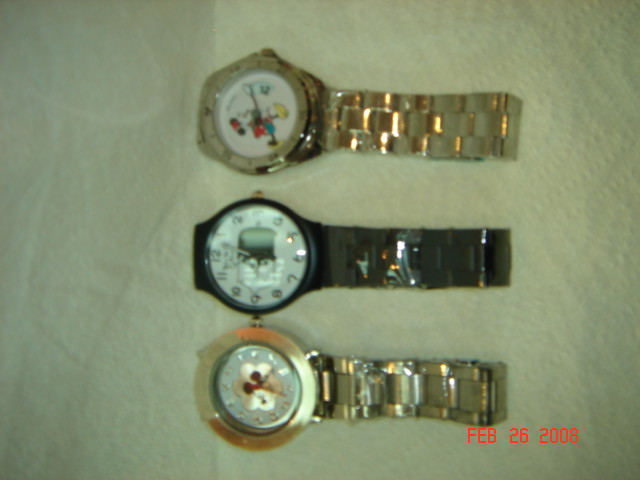This photograph showcases three distinct watches placed side-by-side on a white paper towel. In the bottom right-hand corner, there is red text displaying "FEB 26 2008," indicating the date. 

From bottom to top, the watches are arranged with their clock faces pointing towards the left and their straps extending to the right. 

The first watch at the bottom has a silver band and features a golden clover design at its center. 

The second watch, positioned in the middle, has a black border around its face. The watch face itself is adorned with silver hands and a jade-colored shell design. It sports a dark gray strap. 

The topmost watch depicts a cartoon figure on its face and is predominantly gold in color, including the strap.

Each watch is meticulously arranged to highlight its unique design and characteristics.